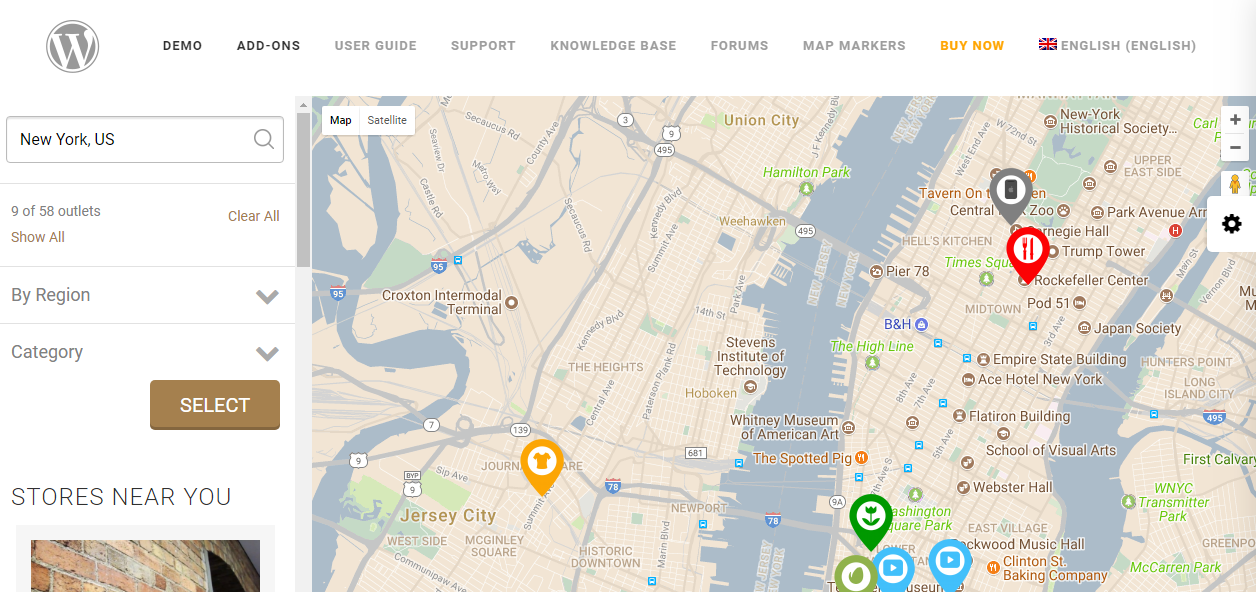Sure, here is a cleaned-up and detailed version of the caption:

---

On the right side of the webpage, occupying approximately one-third of the screen, is a detailed map. The waterways, represented as rivers, are depicted in light blue, while the main streets and land areas are shown in grey. The map highlights seven specific areas of interest related to the user's search results. The header indicates that the map pertains to New York. Below the map, there is a note that mentions nine out of 58 outlets are displayed, categorized by region. Users can select these outlets directly from the map. Additionally, there is a section labeled "Stores Near You."

Higher up on the page, the word "Demos" is prominently featured, with a large, grey-circled capital "W" beside it. The section details demo versions and add-ons, highlighted to catch the user's attention. A bright yellow button labeled "Buy Now" is located further across the page, emphasizing an immediate purchase option. The entire page content is presented in English.

---